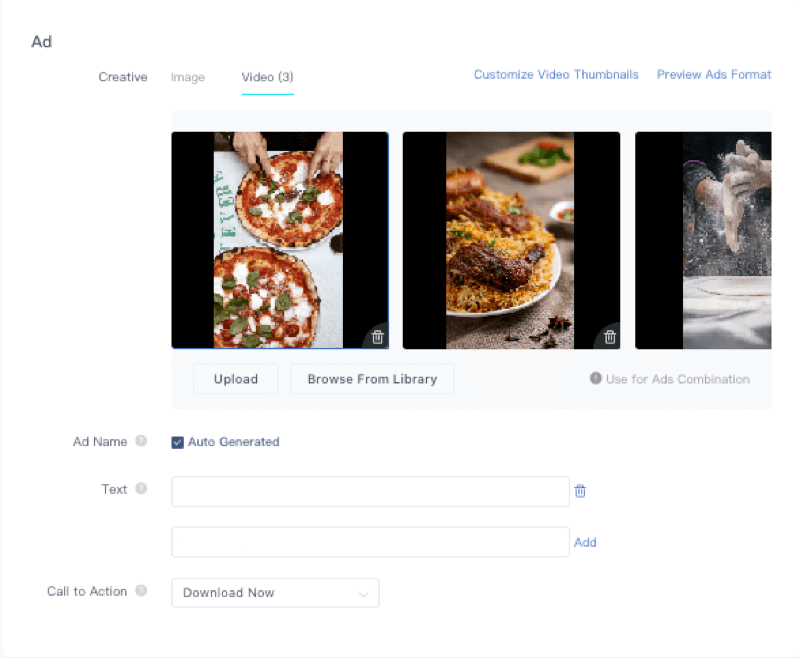The website showcases a series of visually appealing food photographs in what appears to be an advertisement format, indicated by the label "AD" in the upper left-hand corner. There are three striking images, each captured with great attention to detail.

The first image features two pizzas, with one being actively sliced by a pair of hands, suggesting a moment of preparation and anticipation. The second photograph displays a well-composed meal centered around brown rice, topped with what appears to be meat. The background includes a cutting board adorned with fresh greens and slices of bread, adding a rustic touch to the scene. The third image captures the hands of a person dusted with flour, in the midst of an intricate pizza-making process.

In addition to the images, the website offers various customization options highlighted in blue text. These include creative image and video formats, customizable video thumbnails, and preview options. Users can upload their own content, browse from the library, and utilize these elements for ad creation. There is also an auto-generated name feature, a text box for editing, and a straightforward call-to-action button labeled "Download Now," accompanied by a downward arrow for easy access.

Overall, the advertisement effectively combines aesthetic food imagery with user-friendly customization tools, enhancing the appeal and functionality for potential users.